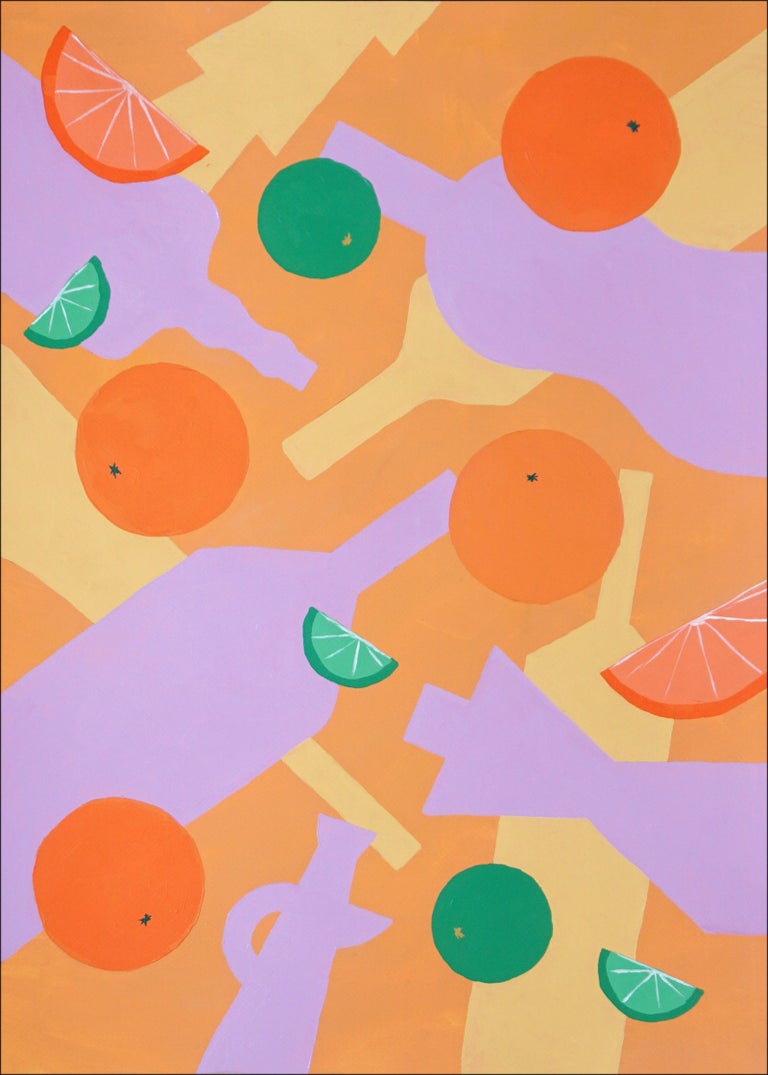This image appears to be a vibrant, computer-generated graphic designed for a bar or alcohol advertisement. The overwhelmingly orange background is adorned with the silhouettes of various bottles, possibly containing champagne, wine, or liquor. These bottles are primarily colored in pale yellow and light purple hues, numbering around nine in total. Interspersed within this backdrop are whole fruits and fruit slices, prominently featuring oranges and limes. Specifically, the image includes four whole oranges and two whole limes, positioned strategically at the bottom left, middle left, upper right, and middle right. Additionally, there are orange slices on the upper left and middle right, and green fruit slices (likely lime) appear in the upper left, center, and bottom right of the image. The oranges have a single black spot indicating the core, enhancing the detail and realism of the floating fruits. This colorful and dynamic composition effectively highlights the theme of refreshment and celebration, making it ideal for a bar setting.